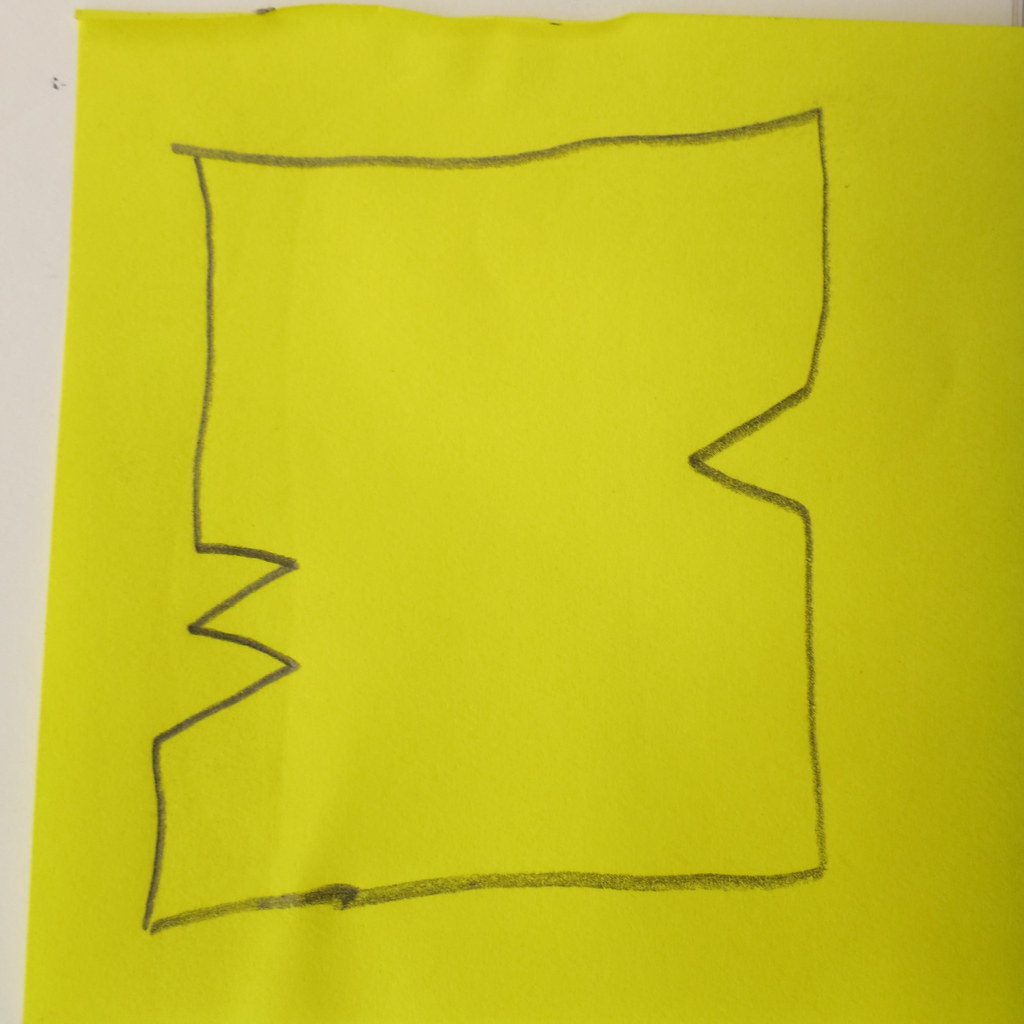The image showcases a meticulously drawn illustration on a yellow piece of paper that is slightly creased and sprinkled near the center. The background is predominantly white, with a streak of grayish-silver running diagonally from the bottom left to the upper left corner, adding depth to the composition. Meanwhile, a gray space frames the drawing above and along the edge.

The focal point of the drawing is defined by a thick, black line that dominates the yellow paper, possibly created with a robust pencil or marker. The line begins at the bottom in a rectangular shape arranged vertically. As it ascends, about a quarter of the way up, the line forms a triangular indention, creating a pointed gap, and is followed by another similar triangular cut-out above it. Continuously extending upwards almost to the edge, the line takes a turn to the right and then descends, incorporating another triangular indent, before extending towards the bottom. This intricate pattern of geometric cut-outs and thick lines contributes to a striking and dynamic visual effect.